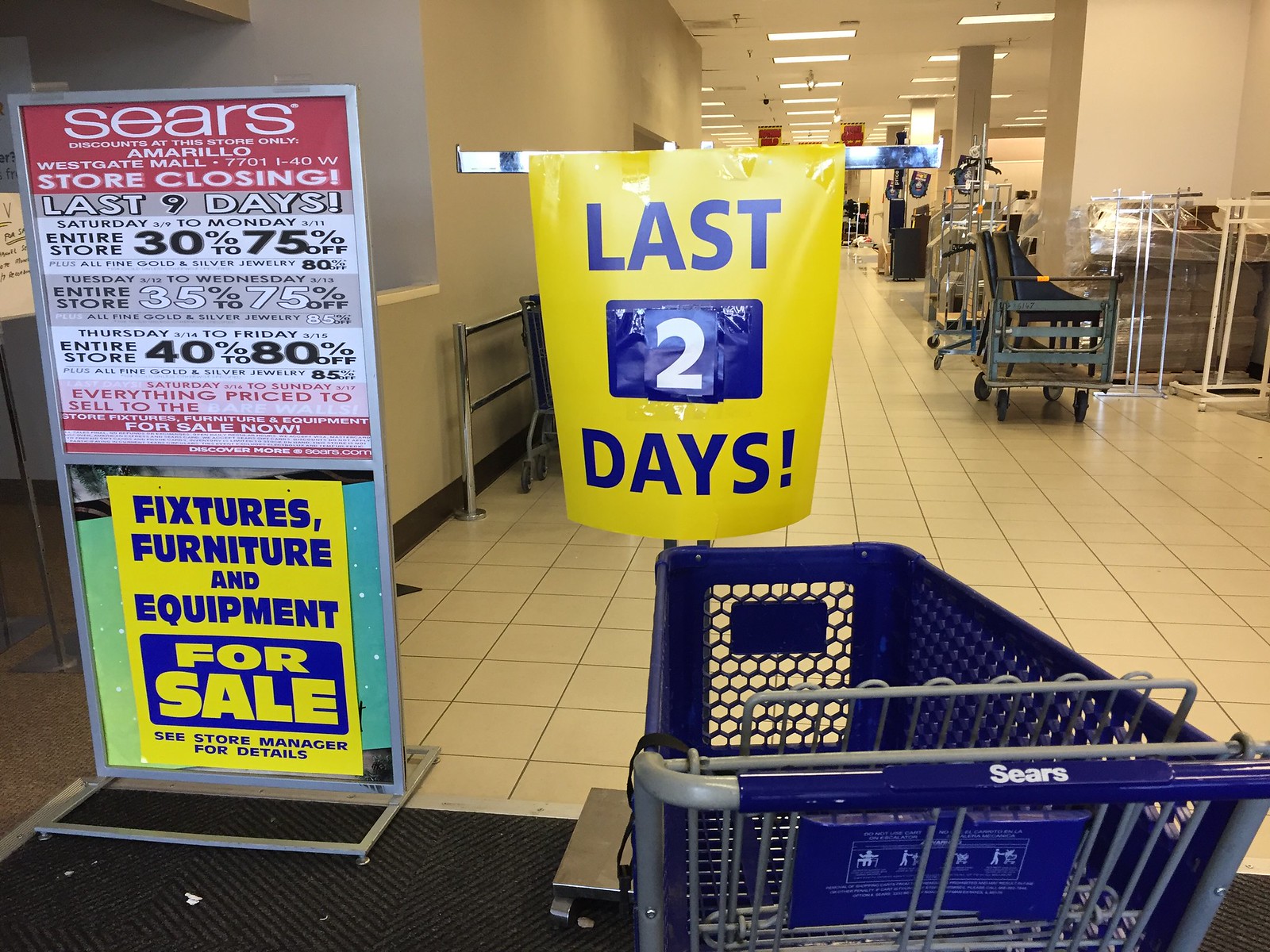Inside a Sears store nearing the end of its operation, a blue shopping cart with a dark blue basket and the word "Sears" prominently displayed on its handle sits in the forefront. The cart rests on a gray, cloth-like rug that marks the entrance area. Directly behind the cart, a large yellow sign with blue text announces, "Last 2 Days," indicating the final days of the sale. To the left of it, a standing advertisement board reads, "Sears Amarillo Westgate Mall Store Closing. Last 9 Days," and lists various percentages off merchandise, emphasizing discounts ranging from 30% to 75% across the entire store. Below this, another yellow sign alerts customers that fixtures, furniture, and equipment are also for sale. The scene extends into the store, revealing a light brown, square-tiled floor and sparse shelving, hinting at the largely emptied space. The store is lightly illuminated by fluorescent lights on the ceiling, while remnants of fixtures and silver metal racks, used for hanging clothes, stand scattered in the background.